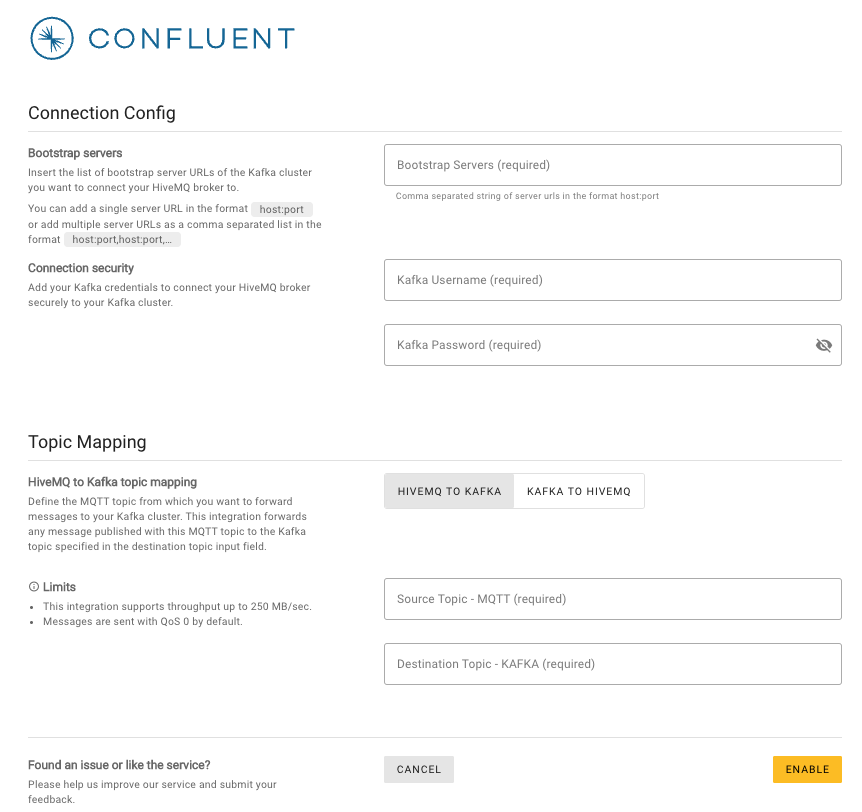The image depicts a section of a website's settings page, specifically an information sheet for connection configuration. In the upper left corner, there is a blue circular icon featuring a crab-like symbol, also in blue. To its right, the label "Confluent" is prominently displayed in uppercase letters.

Below this header, the page primarily consists of black text. The first notable heading is "Connection Config," followed by a subheading specifying "Bootstrap Server" or "Bootstrap Servers," accompanied by additional descriptive information underneath. Further down, the next section is titled "Connection Security," succeeded by "Topic Mapping," and then a sub-section named "HiveMQ to Kafka Topic Mapping."

Adjacent to the "HiveMQ to Kafka Topic Mapping" section is an information icon with the word "Limits" beside it. At the very bottom of the page, a prompt encourages users to provide feedback with the message: "Found an issue or have other feedback? Help us improve our service and submit your feedback."